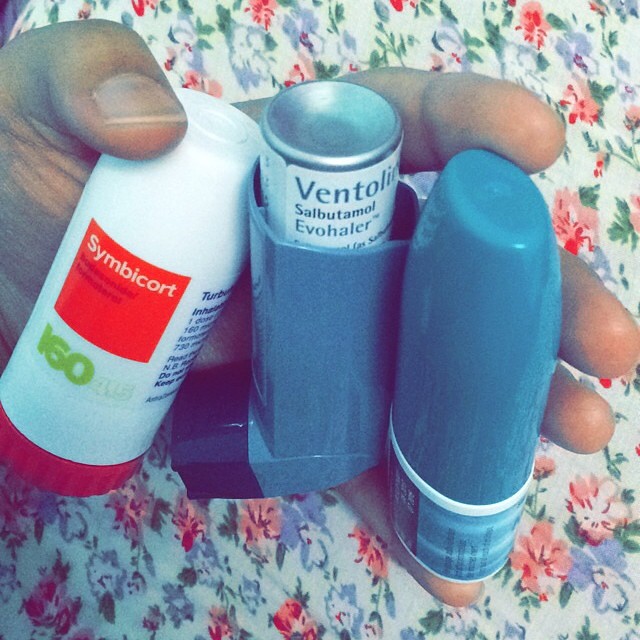The indoor color photograph depicts a Caucasian left hand entering from the left side of the frame and holding three different types of medical inhalers and bottles. The background features a floral print tablecloth. The first item on the left is a white cylindrical container with an orange square label and white text that reads "Symbicort"; it also mentions the dose "ISO 415." The middle item is a gray inhaler with a blue cap, marked "Ventolin," followed by the text "Salbutamol Evohaler." The third item on the right is another cylindrical container with a blue cap and bottom; it might be another type of inhaler or medication, but it's not specified. The hand’s thumb is visible on the left, suggesting it's the left hand holding these items.